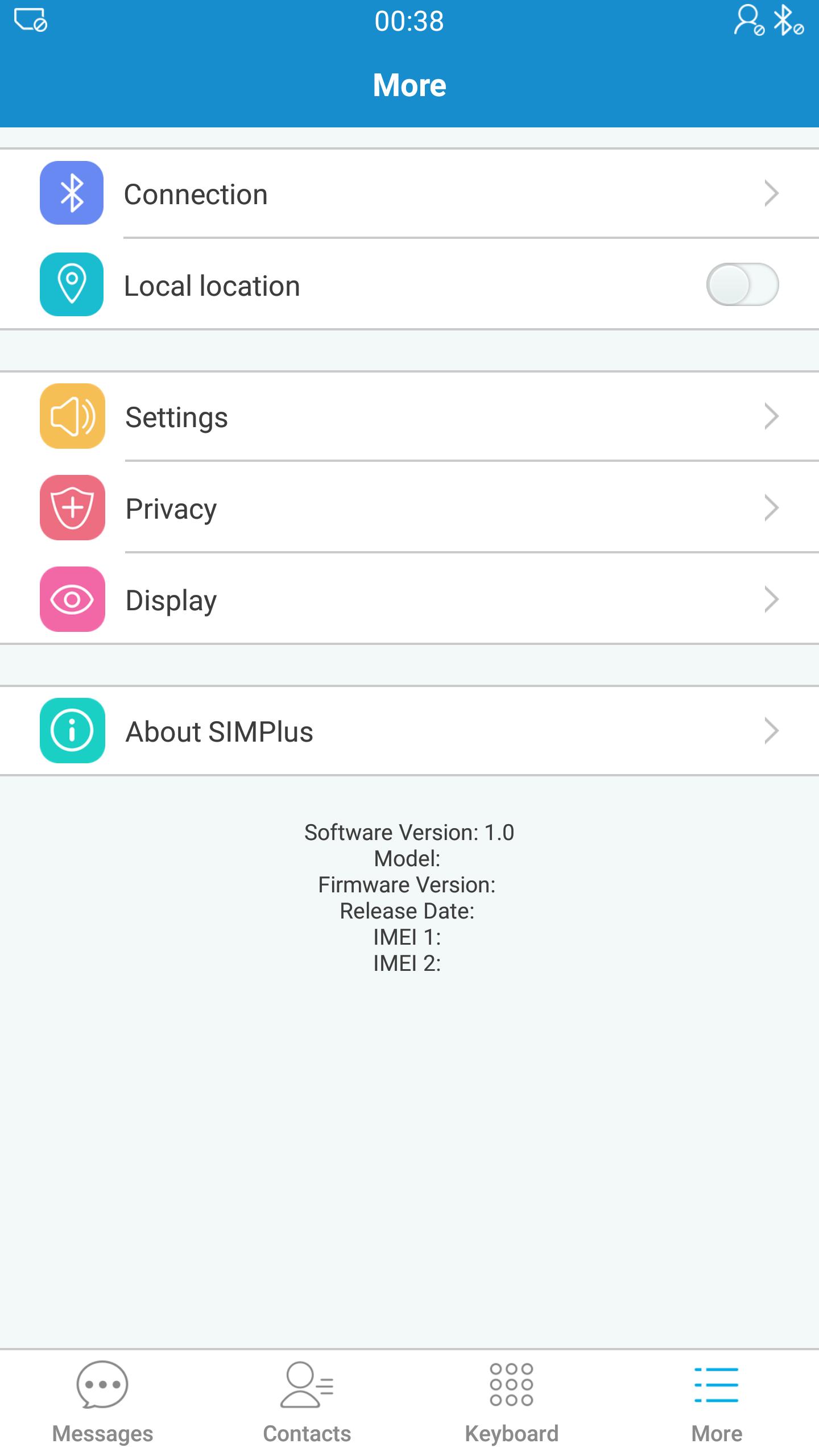This image is a screenshot taken from a phone, showcasing its settings page. At the very top, there's a blue banner featuring indicators for the time (00:38), Bluetooth, and user account. Below the banner, there are several setting options displayed, including "Connection," "Location," "Settings," "Privacy," "Display," and "About CIDM Plus." Following these options, the page provides technical details such as "Software Version 1.0," "Model [blank]," "Firmware Version [blank]," "Release Date [blank]," "IMEI 1 [blank]," and "IMEI 2 [blank]."

Further down, there are buttons for "Messages," "Contacts," "Keyboard," and "More." The entire page is presented on a plain white background, with each category highlighted in a brighter white and accompanied by black text. Icons are designed in a curved square style and come in various colors, including blue, teal, yellow, red, and pink. The layout is in a vertical portrait orientation, typical for a phone. Although additional context is lacking, it appears to be a settings page specific to the phone itself.